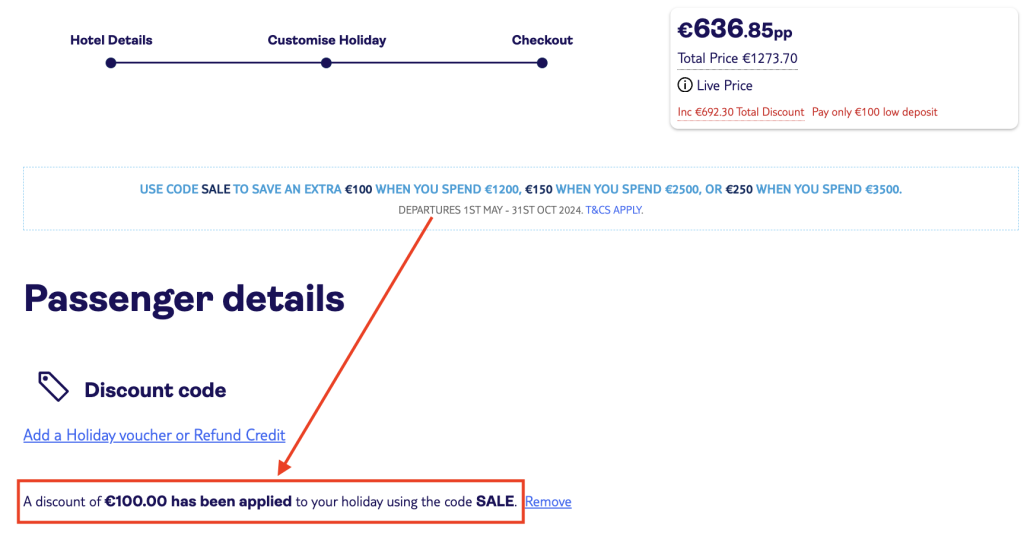This image appears to be an advertisement or screenshot for a hotel booking service, set against a white background. 

At the top left, there is a navigation line with three sections, each accompanied by a dot: "Hotel Details" on the far left, "Customize Holiday" in the middle, and "Checkout" on the right. To the right of this navigation line, there is a gray-outlined box displaying the price information. It lists the price as £636.85 per person and the total price as £1273.70, indicating the currency is in British Pounds.

Beneath this price information, there is a circle with an ‘i’ inside it labeled "Live Price." Below that, in red text, it states, "Included: £692.30 total discount. Pay only £100 low deposit."

Further down, a rectangular banner reads, "Use Code 'SALE' to save an extra £100 when you spend £1,200, £150 when you spend £2,500, or £250 when you spend £3,500. Departures between 1st May and 31st October 2024. T&C's apply."

A red arrow points downward to the bottom of the screen, where there is a prominent red rectangle that declares, "A discount of £100 has been applied to your holiday using the code SALE."